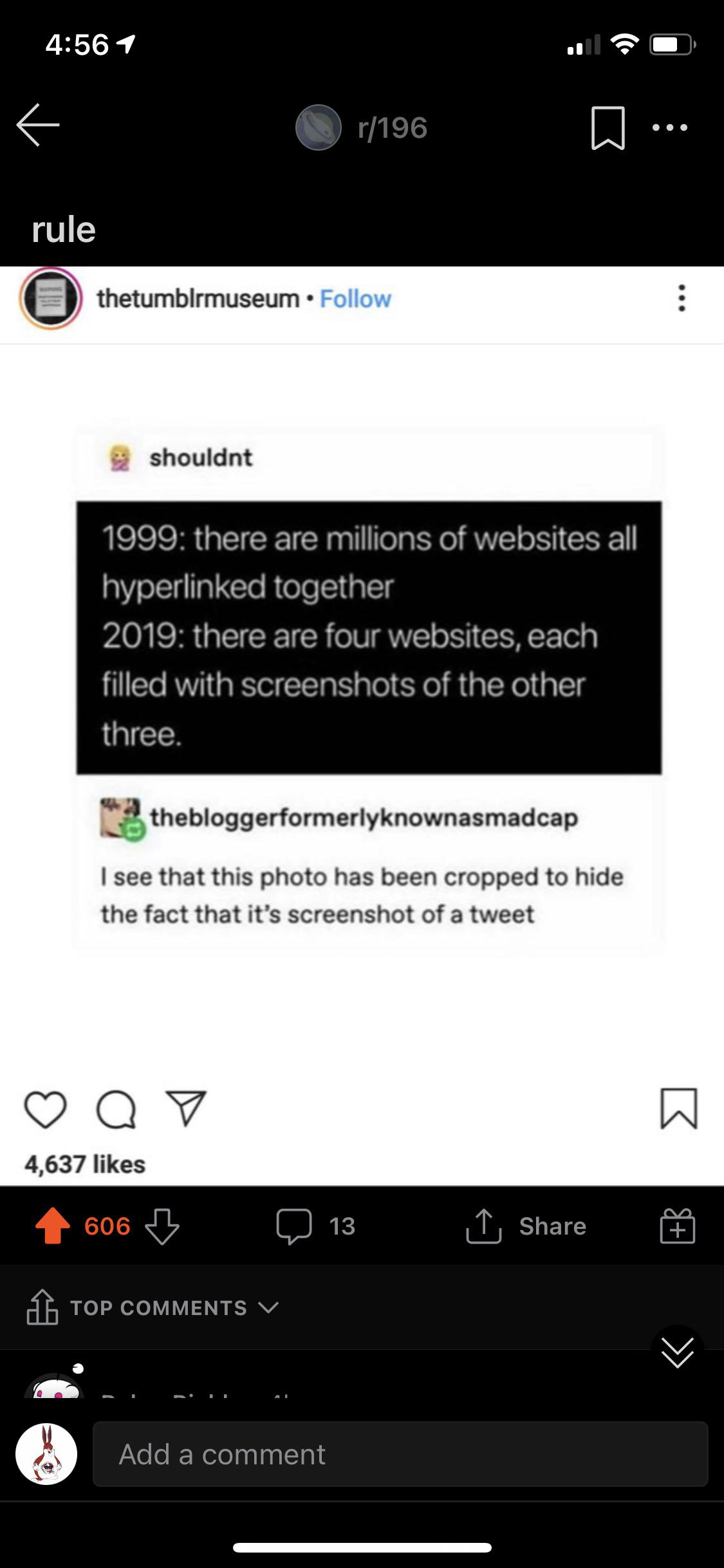The image shows a screenshot of a cell phone's screen at 4:56 PM. Located in the top-left corner are the current time and, to its right, a series of status icons including a connection signal, a Wi-Fi icon, and a battery percentage bar. Directly beneath these icons is a navigation bar featuring an "R/196" label, a left-pointing arrow, a bookmark icon, and three vertical dots.

Below the navigation bar, the image features a user interface section with a black background that states, "Tumblr museum" in blue text, suggesting an option to follow, accompanied by a rule. Following this, the text reads, "In 1999, there were millions of websites all hyperlinked together. In 2019, there are four websites, each filled with screenshots of the other three."

Further down, there's a comment from "the blogger formerly known as Madcap," highlighting that the photo has been cropped to hide that it is a screenshot of a tweet. This section has a white background and shows a substantial amount of engagement with 4,637 likes.

At the bottom of the screen, there's a black interface bar displaying 606 upvotes in orange, 13 comments, and a share icon. Beneath these elements, top comments can be viewed, followed by the option to add a comment, indicated by a white circular profile picture of a Reddit character. The screen ends with a white horizontal line in the center at the very bottom.

The layout of the image demonstrates a typical social media interface, showcasing the interplay of different platforms and the interconnectedness of web content.